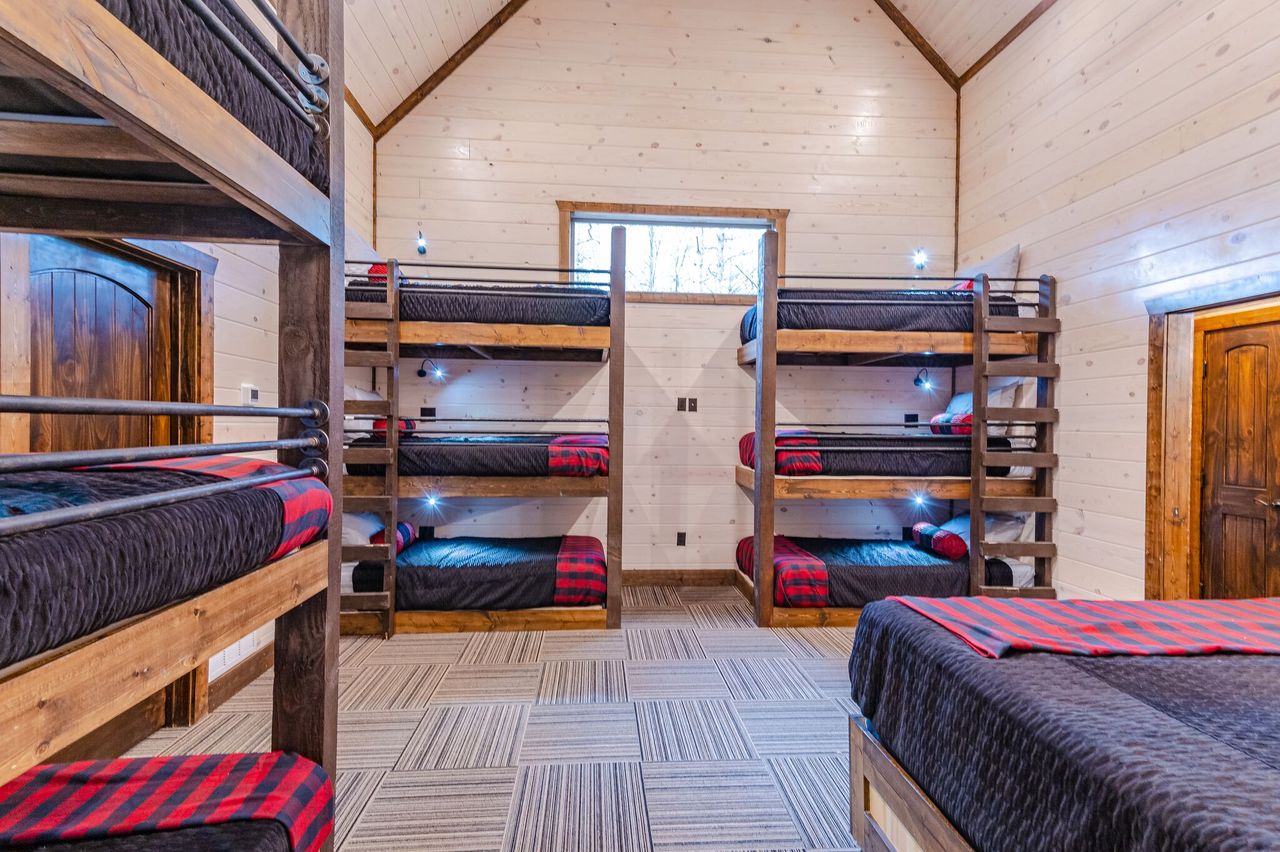The image depicts an intriguing bedroom, possibly in a children's camp. The room features a total of ten beds: nine in the form of three sets of three-story bunk beds and one queen-size bed. The left side of the room hosts the first set of three-level bunk beds, while the back wall contains two more sets, with matching dark bedspreads and striped red and black blankets at the ends of each bunk. Each bunk includes safety railings made of three metal rods. 

The queen-size single bed is positioned on the right side of the image. The room, which is captured during the daytime, is illuminated by natural light seeping through a rectangular window on the back wall, situated at the level of the top bunk. The walls, built from light-colored wood slats, contrast with the darker wooden doors located at the center of both the left and right sides.

The floor exhibits a unique pattern of light brown, alternating in vertical and horizontal rectangles. The room also features electrical sockets on the central back wall between the sets of bunk beds. These details suggest a practical yet aesthetically harmonious design in the context of a cozy and methodically structured sleeping area.